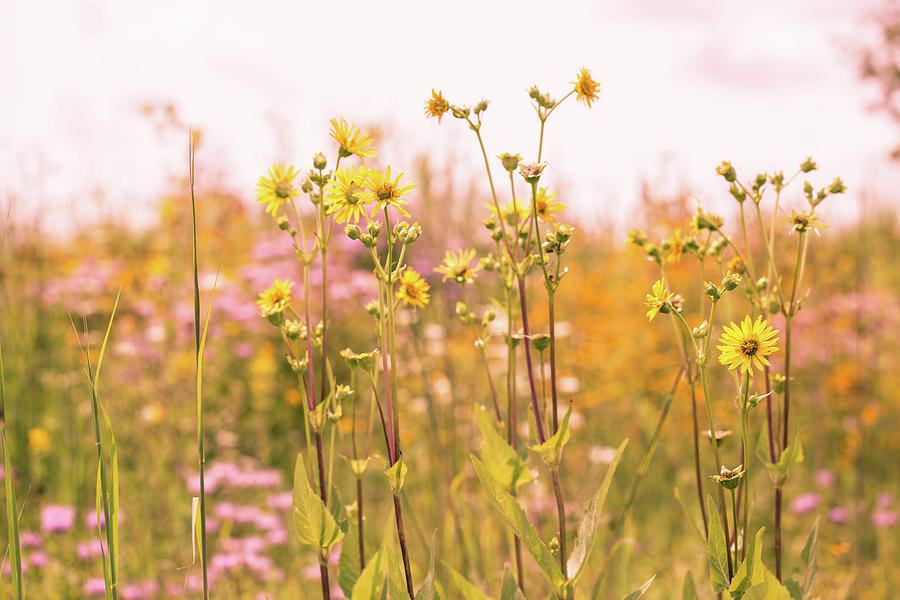The image captures a serene field of tall, yellow wildflowers with thin green stalks and sparse leaves, standing prominently in the foreground. Each stalk bears multiple flowers along with bulb-like buds, some of which are slightly or fully opened, showcasing yellow petals with a center that is a mix of black and yellow or occasionally orange. The main flowers are in sharp focus, providing a detailed and clear view, while the background remains blurry, suggesting a vast expanse of flowers in pink, orange, and yellow hues, accompanied by green foliage. The sky is overcast with a white or hazy purple-pink tint, which might suggest clouds, enhancing the moody atmosphere. The image, though not vividly colored and somewhat aged in quality, is well-lit, indicating it was taken during the day. Adding to the depth, vague outlines of rocky cliffs can be perceived in the distant, blurred background, contributing to the natural and tranquil setting of the scene.